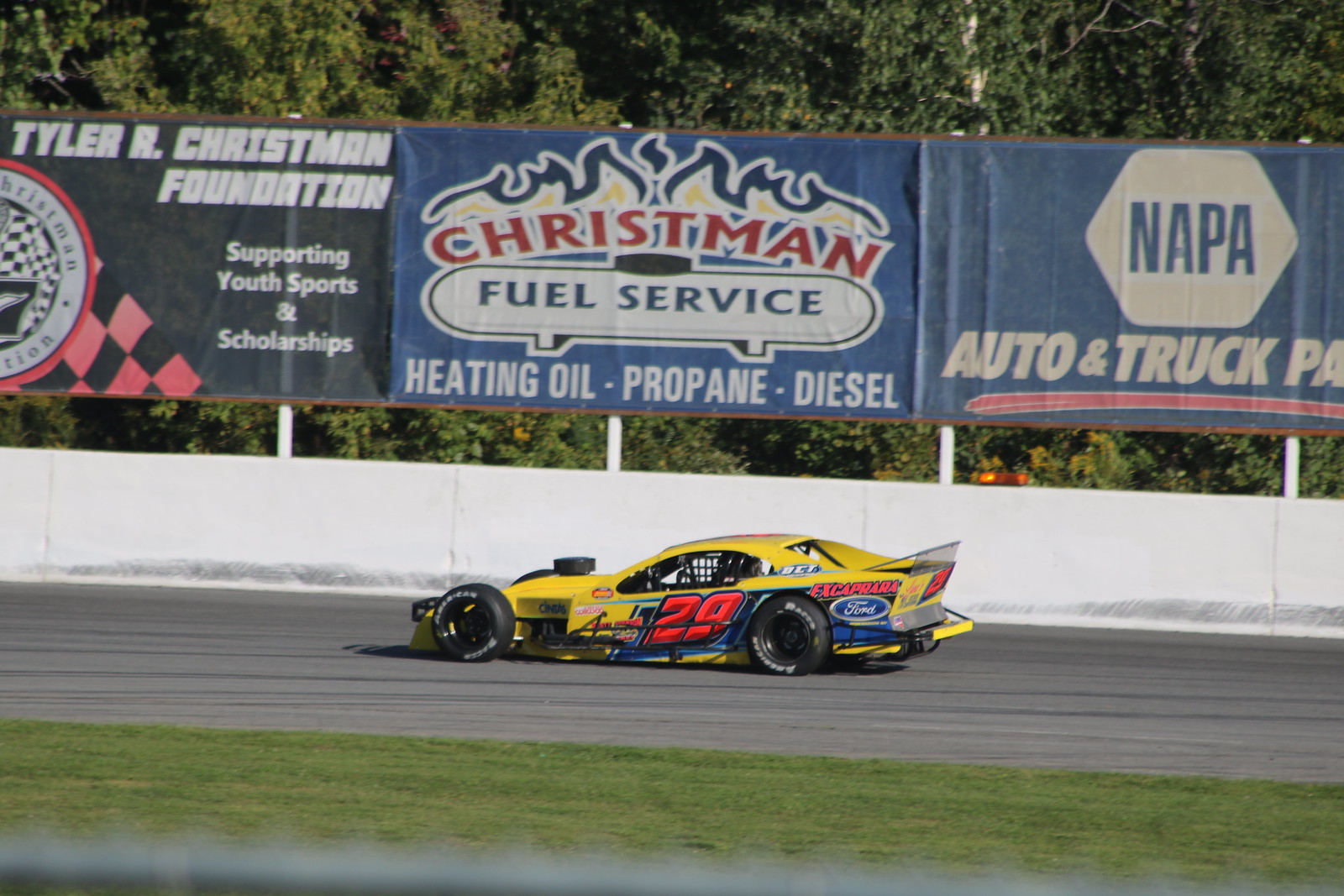In the forefront, a green field of grass stretches horizontally across the bottom of the image. Just beyond the grass lies a medium gray racetrack with black streaks. Bordering the racetrack is a white safety wall smeared with tire marks at its base. Above the wall are three distinctive signs. On the left, the sign reads "Tyler R. Christman Foundation, supporting youth sports and scholarships" in white font on a black background, with a seal flanked by black and pink checkered bands. The middle sign states "Christman Fuel Service, heating oil, propane, diesel" in red and blue with flames emanating from the lettering. The third sign, on the right, says "Napa Auto and Truck Parts," featuring a white hexagon with "Napa" inside and a red streak beneath the text. In the center of the image is a yellow race car marked with the number 29. The car features several logos, including one that reads "X Caprera" above a Ford symbol near the back tire. The backdrop includes green trees and shrubs, completing the scene.